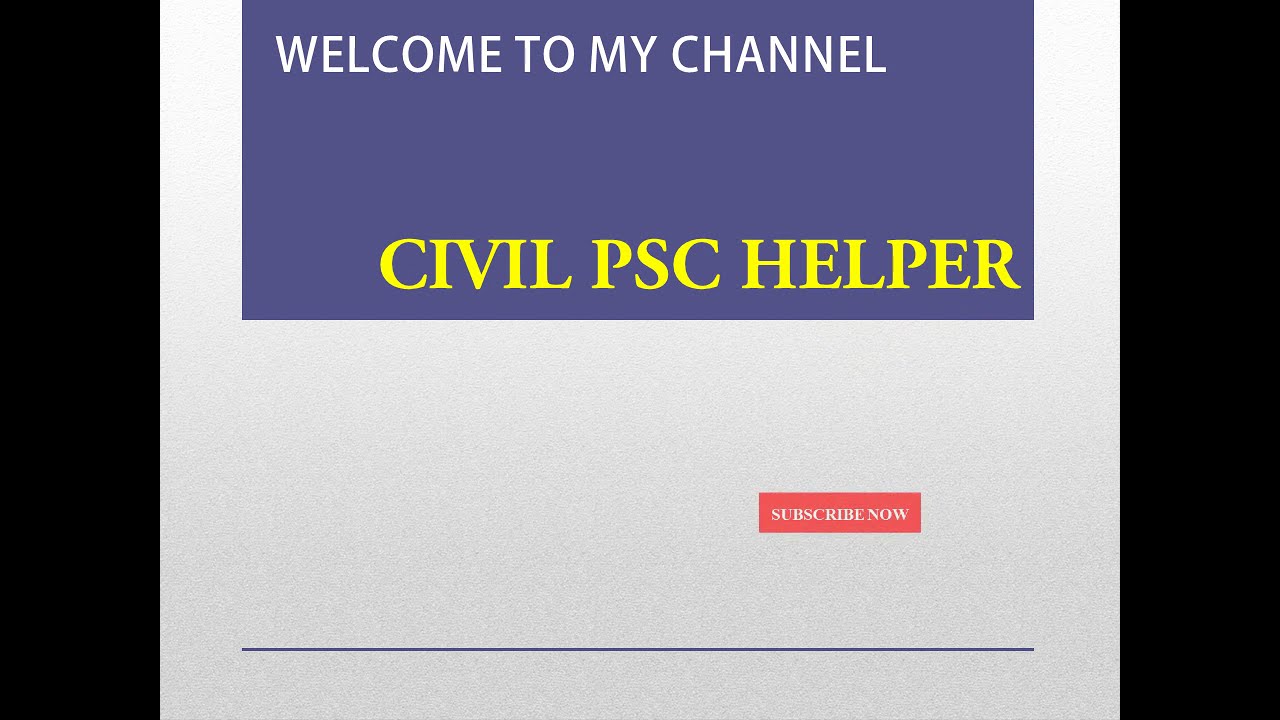The image depicts a structured banner that appears to be designed for a YouTube channel. It features a slightly textured, almost white background framed by large black borders on both the left and right sides, occupying roughly one-eighth of the total width each. Prominently positioned near the top is a smaller, purple rectangle containing the text "Welcome to My Channel" in white letters. Directly beneath this, in bright yellow text, is the phrase "Civil PSC Helper". Towards the bottom middle section, there is a small orange rectangle with white text that reads "Subscribe Now". Finally, a thin blue line stretches horizontally across the very bottom of the image, adding a stylistic touch to the overall composition.